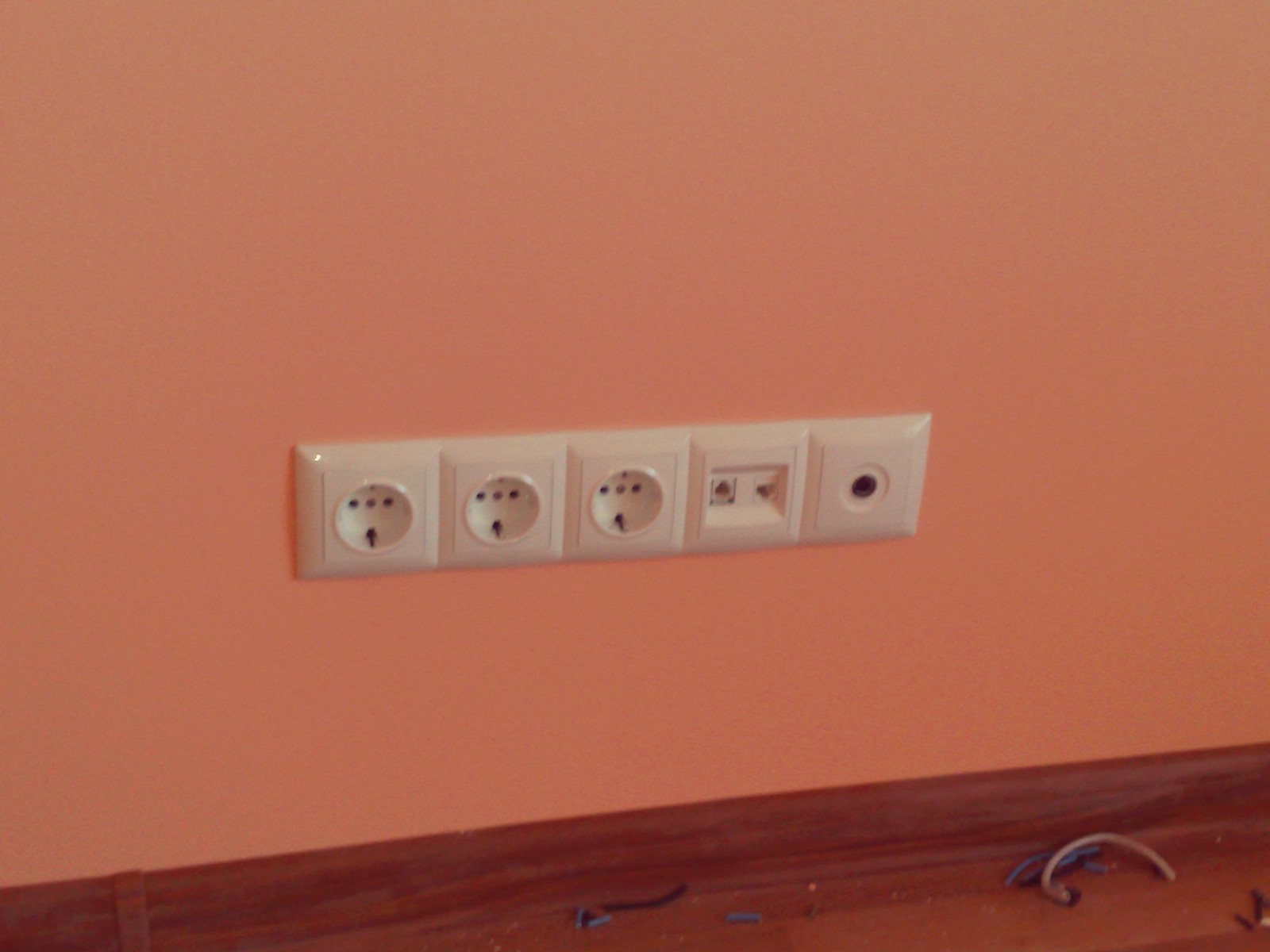This detailed photograph showcases a horizontal alignment of five off-white electrical outlets on a pale orange wall, characterized by its melon hue. Below the outlets is a dark brown, wood-like trim that runs horizontally, acting as either a baseboard or the edge of a counter. This trim is cluttered with what appears to be debris, including several clipped electrical wires in different colors such as light blue, black, and light gray, which lay haphazardly along the wooden lip.

The five square-shaped outlet panels in the image are distinguished by their varying designs. The first three outlets from the left feature large circular indents housing three small holes arranged in a triangular pattern, with an additional slit at the bottom. These unusual configurations suggest they might be specific to certain regions, possibly in Asia. The fourth outlet shifts in design, presenting two square openings that might accommodate specific plugs, likely different from the previous ones. The fifth and final outlet on the far right contains a distinct double circle with a central hole, resembling a large black button, possibly for a reset function or breaker switch.

The collective presentation of the outlets, wires, and the distinct color contrast between the wall and the trim contribute to the overall visual intricacy of the image.